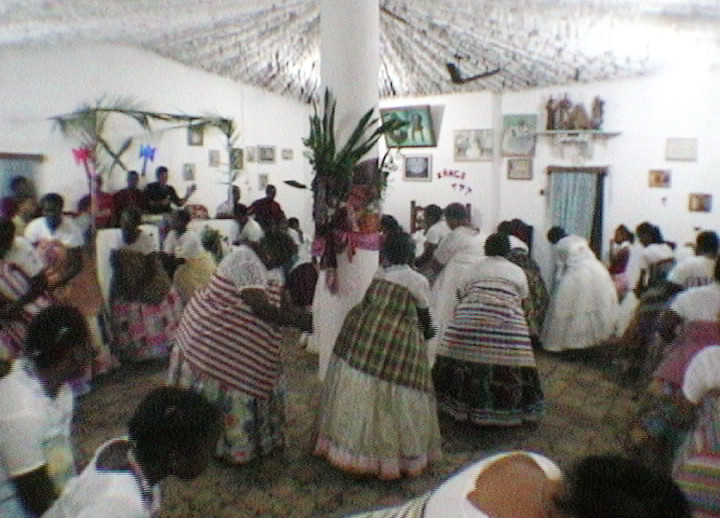The image depicts a vibrant festival scene within a white-painted room adorned with numerous pictures, paintings, and ornaments. Central to the picture is a tall white pillar, approximately 10 to 12 feet high, draped with colorful cloths and greenery, such as palm fronds and a flower wreath around the middle. Surrounding this pillar, a group of African American women dressed in ornate white dresses and patterned, colorful shawls and wrappers are seen dancing and moving in circles with their heads bowed, possibly in a form of prayer or celebration. Their attire features a mix of dusty colors like red, white, green, yellow, orange, and blue, with some fabrics displaying striped patterns. The ground is a multicolored patterned floor, adding to the festive atmosphere. In the background, a curtain hangs in a doorway, and to the left of the pillar, there is a stand constructed from tree limbs, where two or three men sit, slightly elevated, observing the proceedings. The combination of the women's vibrant clothing and the richly adorned room creates a lively and celebratory ambiance.